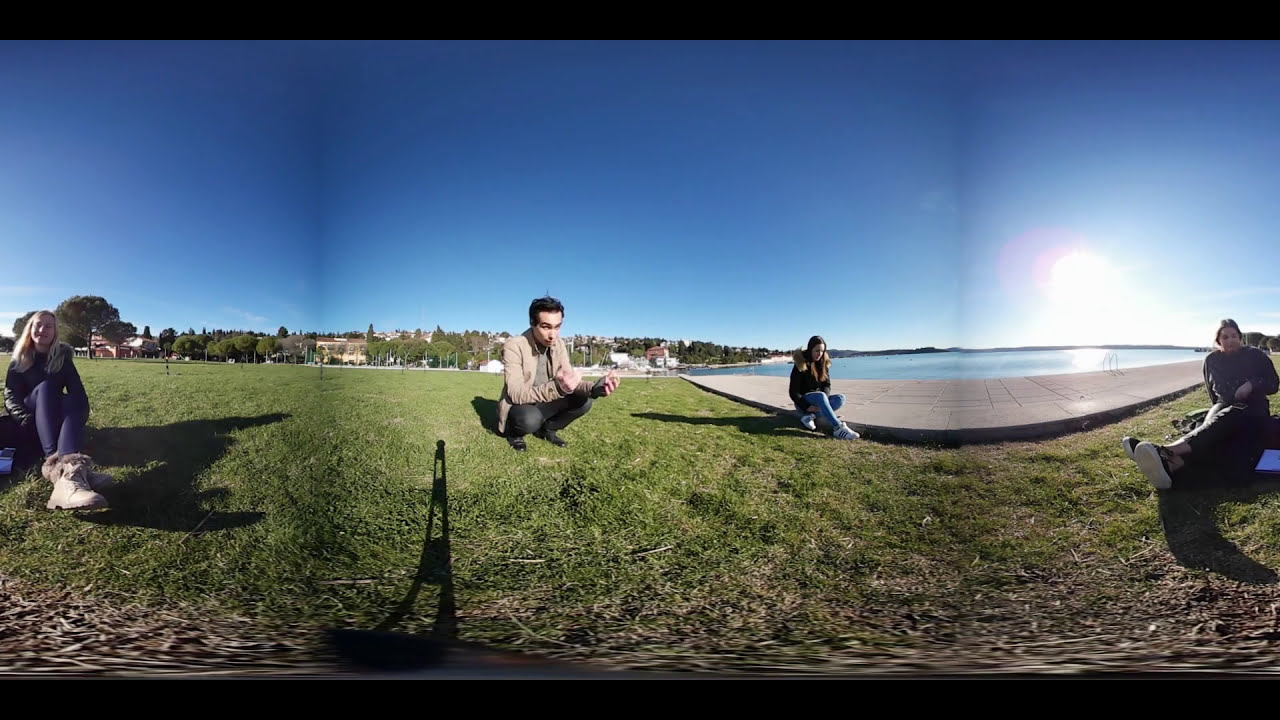In this panoramic photo capturing a crystal clear blue sky, a group of four people are seen relaxing in a park. They're seated on a grassy field that stretches to the left side of the image, with a bit of a dock leading towards a body of water visible behind them. The horizon reveals a thin tree line and distant houses. 

On the left, a woman wearing purple pants and a black jacket with shoulder-length blonde hair sits with her left leg crossed over her right, smiling at the camera. Next to her, near the center, a man with short black hair and pale skin is squatting low, dressed in black pants and a brown jacket, his elbows resting on his knees, with fists formed and facing upwards. 

Further to the right, another woman with brown hair is seated on the pavement right beside the grassy field, her left leg bent across her body under her right leg, which extends forward. She sports a black jacket with fur trim around the neck. The rightmost person is a woman with dark blonde, head-length hair, sitting with both legs stretched out in front of her, her left leg crossed over the right, twisting slightly to look at the camera. 

In the background beyond the pavement, there's a glistening body of water, completing the serene park setting.